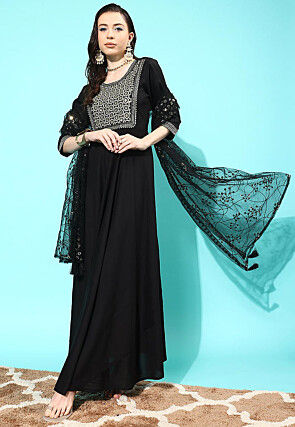The full-color, vertically rectangular photograph, taken indoors under artificial lighting, features a staged scene against a plain aqua blue wall background. In the image, a woman stands just left of center, occupying most of the vertical space. She has long dark hair and fairly light-colored skin, suggesting she might be Caucasian. She is dressed in a floor-length black dress with sleeves ending below her elbows, accompanied by a black shawl draped over her shoulders. Silver earrings adorn her ears. Her hands are clasped just above her hips, and she is barefoot, with one foot slightly forward. Her serious expression gives her a no-nonsense appearance. A pronounced shadow from the lighting is cast on the blue wall behind her and the brown and white grid-patterned floor beneath her.